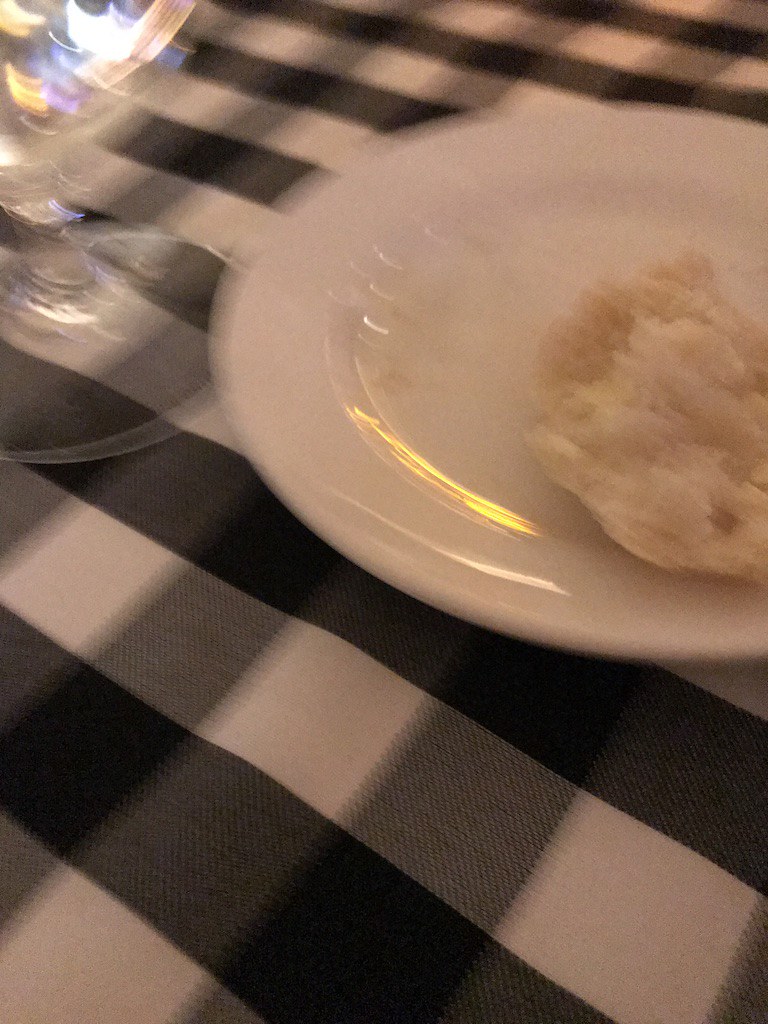A blurry and low-quality color photograph captures a table setting adorned with a black and white checkered tablecloth, where the colors blend together into shades of gray. Dominating the scene is a white, opaque ceramic plate, positioned toward the right-hand side, featuring a solitary piece of bread or possibly an uncooked half of an English muffin. Light reflections dance across the scene, notably bouncing off a crystal goblet located to the left of the plate, casting shimmering glints onto the tablecloth and creating additional highlights on the plate itself. The dark and light stripes of the tablecloth, featuring subtle vertical light gray lines, add a textured plaid pattern, contributing to the intricate yet indistinct composition.